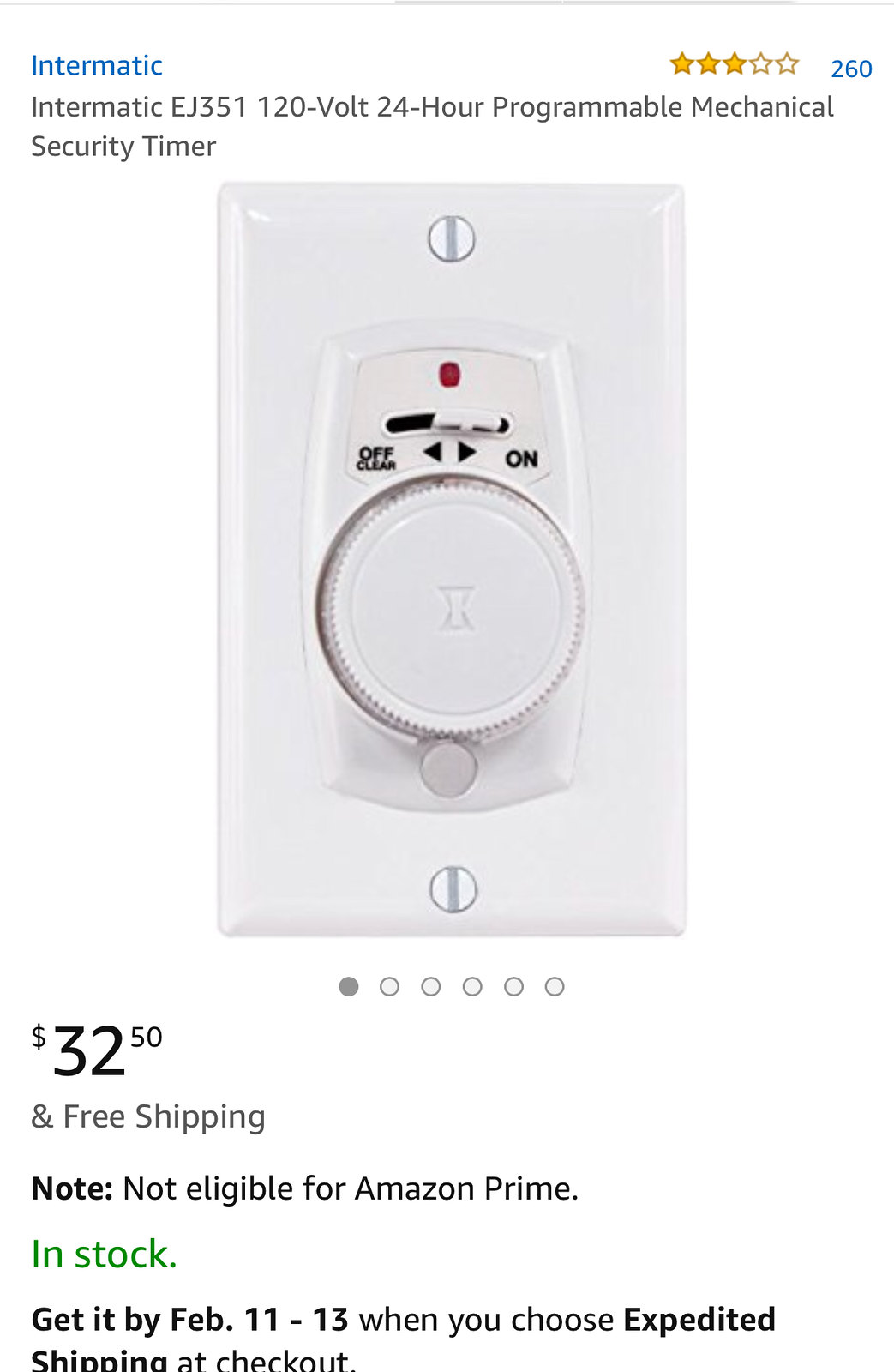Here's a refined and detailed caption for the described image:

"This screenshot from an Amazon.com store page features the Intermatic EJ351 120-volt 24-hour Programmable Mechanical Security Timer. At the top of the page, the brand name 'Intermatic' is prominently displayed in blue font. Below this, the product name 'Intermatic EJ351 120-volt 24-hour Programmable Mechanical Security Timer' is listed. On the upper right corner, the item has received a rating of three out of five stars, depicted by three filled yellow stars and two empty stars, with the total number of reviews marked as '260' in blue font. The main section of the screenshot displays a clear image of the product, which is a timer designed to attach to a light switch. The timer features a rotating bezel to set the timer and has an 'off' position marked as 'Off Clear' with an option to switch it to 'on' using a white tab. Below the image, the price is listed as '$32.50,' with information below indicating 'and free shipping.' However, it is noted that the item is 'Not eligible for Amazon Prime.' In red, it is clearly stated 'In Stock.' Additional shipping information is provided, suggesting that with expedited shipping, the item can be delivered by February 11-13."